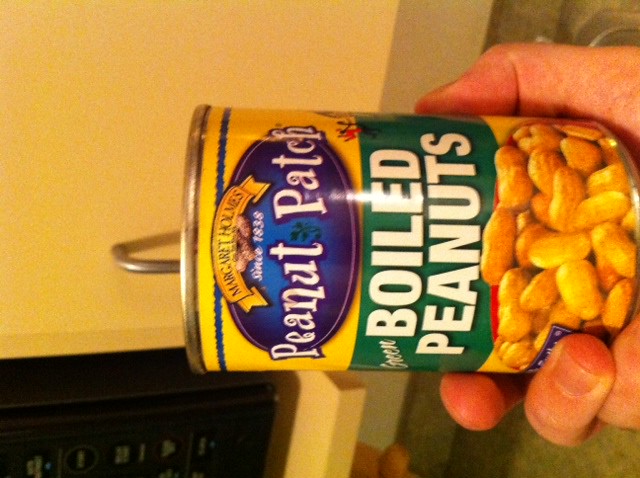In this photograph, a right hand holds up a can of boiled peanuts, prominently displayed against a kitchen backdrop featuring a wooden cabinet and a black microwave. The can itself boasts a vibrant yellow label, with a striking green stripe running horizontally through its middle. Across this stripe, "BOILED PEANUTS" is boldly printed in white, capital letters. Positioned above this text is a blue oval containing "Peanut Patch" written in white font. Crowning the design is a yellow banner inscribed with "Margaret Holmes." Below the bold "BOILED PEANUTS" text, there's a vivid photographic image of boiled peanuts nestled in a red bowl. Interestingly, the entire image has been rotated anti-clockwise, presenting what was originally a portrait-oriented photo on its side.